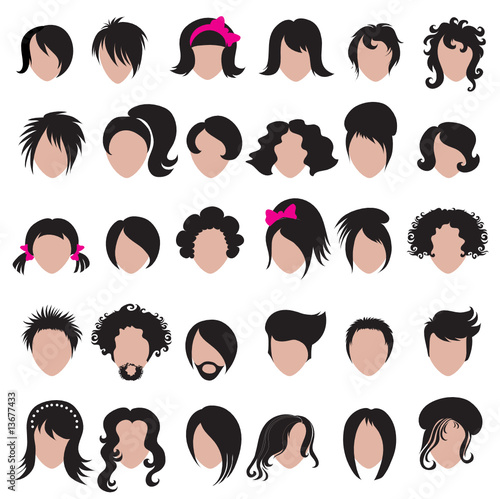The image depicts a grid of simplified, cartoonish human heads, organized in six columns and five rows, resulting in 30 heads in total. Each head is a faceless beige oval, pointed at the bottom where the chin would be, and features diverse black hairstyles, ranging from short curly hair to long wavy hair, ponytails, updos, frizzy hair, and pigtails. A few of the heads are adorned with pink accessories, such as bows or a headband. Notably, one head in the top row and another in the third row down have pink decorations. The hairstyles indicate both male and female representations, with some even featuring beards. The background is white, and the bottom left corner bears the text "Adobe Stock" in small, vertically arranged black print, accompanied by a number.